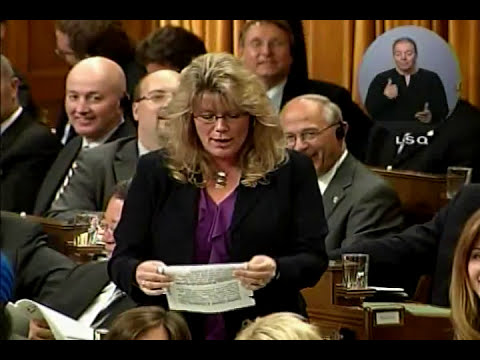This photograph captures a Canadian politician, believed to be Shelley Glover, standing and reading from a sheet of paper in what appears to be Parliament or a council meeting. She has long, blonde, slightly puffy hair and thin, black-framed glasses. Shelley is dressed in a purple blouse beneath a black blazer, accessorized with a necklace and a couple of rings on her fingers. 

The setting is an indoor auditorium, with other members of Parliament or speakers visible seated behind her, all in business attire including grey and black blazers, ties, and some with cups of water in front of them. The men behind her seem to be engaged in laughter or smiles, though it's uncertain if it’s directed at her or with her. Additionally, a sign language interpreter is superimposed in a circle at the top right corner of the image, visually representing the notes being read. The scene is framed with wood paneling on the wall to the left, adding a formal aesthetic to the setting.